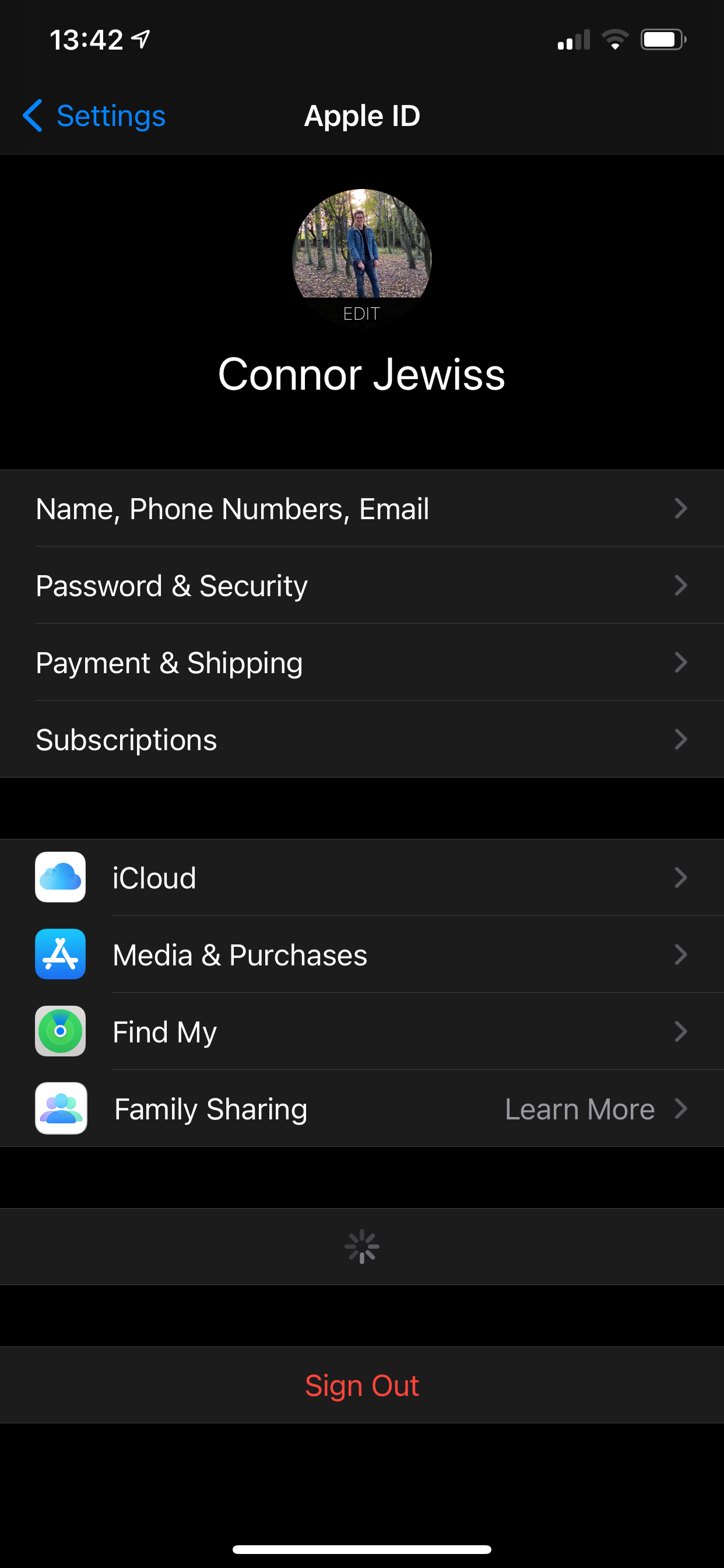This is a detailed caption for the given voice description of the image:

"A screenshot of an Apple ID settings screen on an iPhone in night mode. The background of the screenshot is entirely black. At the top center, the text 'Apple ID' is displayed, below which there is a large, round profile photo. Underneath the profile picture, the name 'Connor Jewess' appears prominently in large white letters. Following the name, four options are highlighted in separate lighter black boxes: 'Name, Phone Numbers, Email,' 'Password and Security,' 'Payment and Shipping,' and 'Subscriptions.' 

Below these options is another lighter black section containing additional settings: 'iCloud,' 'Media & Purchases,' 'Find My,' and 'Family Sharing.' There is a space below this section, followed by a thin lighter black bar featuring a loading icon in the center. Further down, after another space, there is a lighter black bar with the word 'Sign Out' prominently centered in red text."